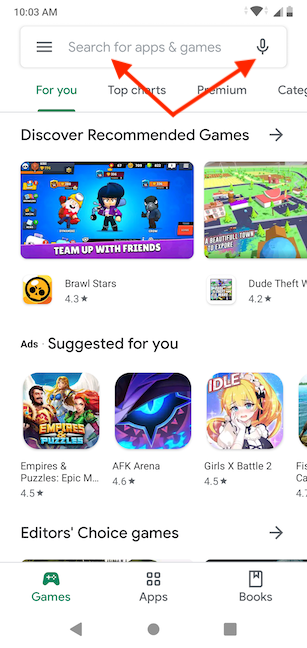The image depicts a smartphone screen with a white background. At the top, the time reads "10:03 AM" accompanied by various status icons. Below this, there is a search bar with a gray background and three horizontal lines inside it. The search bar contains the text "Search for apps and games" and a microphone icon on its right end. 

Two large red arrows converge at the bottom of the search bar; one arrow points to the word "search" and the other points to the microphone icon. Underneath the search bar, there is a blue, underlined text reading "For You," followed by tabs labeled "Top charts," "Premium," and another partially visible word. Further below is a line dividing the sections and the text "Discover recommended games" with a right arrow next to it.

The image showcases two games prominently: "Brawl Stars," which features an image of a yellow box with a circle containing a skeleton head with black eyes and has a rating of 4.3 stars, and "Dude Theft Wars," with a rating of 4.2 stars. Following this is a small box labeled "Ads" and the tagline "Suggested for you."

Additional games listed include "Empires & Puzzles: Epic Match 3" with 4.5 stars, "AFK Arena" with 4.6 stars, and "Girls' Frontline" with 4.5 stars. There is a partial view of another game, the name of which isn't fully visible. 

Below this section, there is a header reading "Editor's Choice Games" accompanied by a dividing line and a right arrow. At the bottom of the screen, the tabs "Games," "Apps," and "Books" are visible in green. The navigation bar at the base of the screen features a left arrow, circle, and square icons.